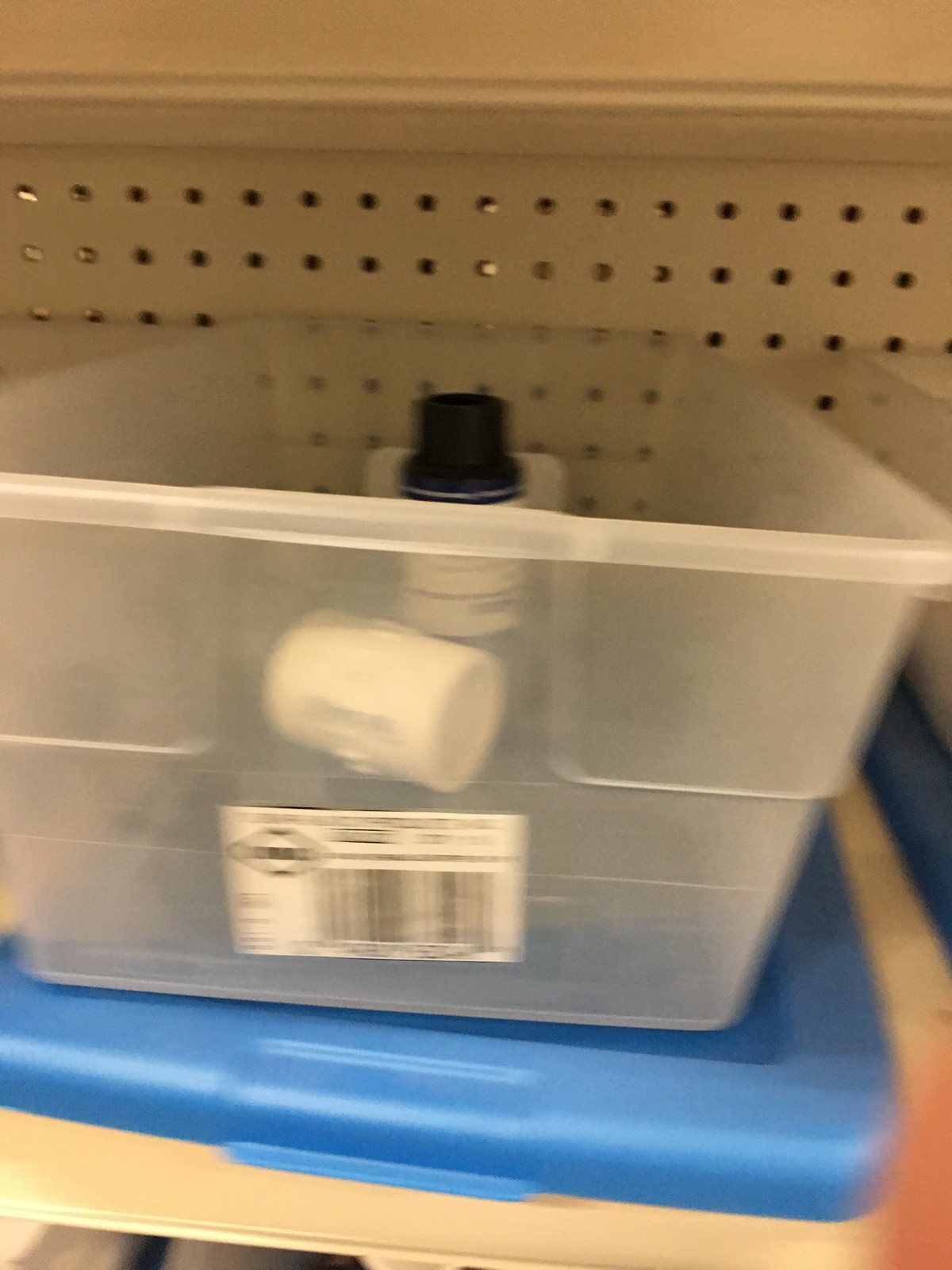In what appears to be a hastily taken photograph, two Rubbermaid containers are situated on a shelf with a pegboard backing, resembling display shelving in a store. The upper container is open, while the bottom one is sealed with a blue lid. Both containers seem to contain substances that resemble drugs. A barcode label is affixed to the side of the bottom container, but the text is unreadable due to the rushed nature of the photograph. Additionally, a bottle lies on its side next to the containers. It appears to have a blue body with a large white label and a black screw-on cap, though details are difficult to discern. Partial edges of more containers are visible to the side, but no further details can be made out.